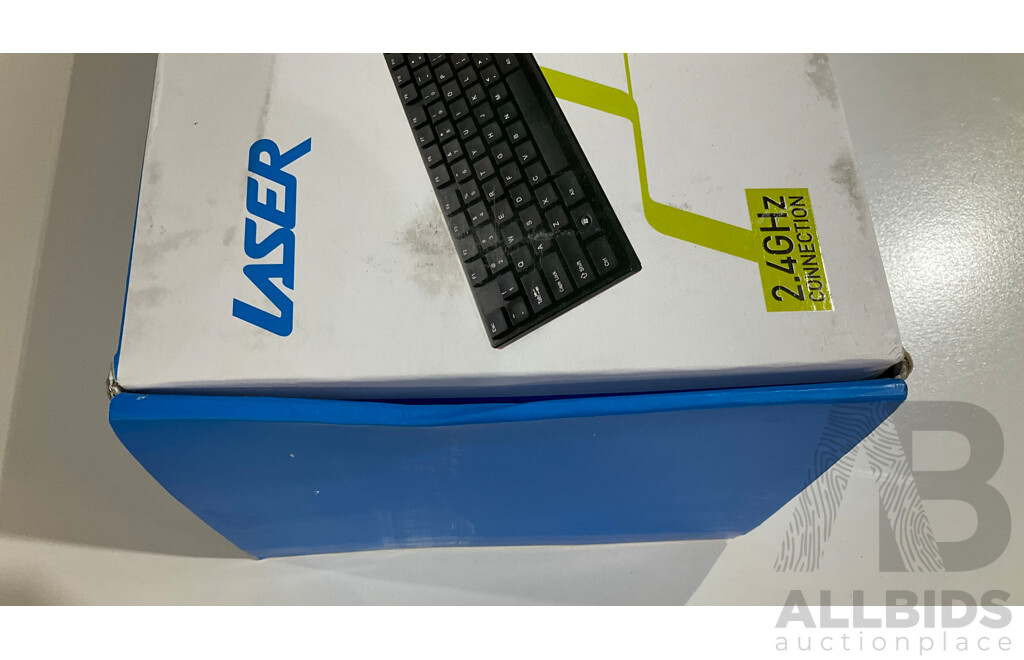The image is a close-up photo of a box placed on a surface with a background that appears to be either white or light gray, likely a floor, table, or desk. The visible side of the box occupies the lower part of the photo, showcasing its blue color. The top of the box is partially visible, displaying the word "laser" in blue text oriented sideways due to the angle of the image. A cut-off image of a black keyboard with white lettering is also visible on the top of the box, accompanied by a stylized design in a yellowish-green color. A sticker located in the bottom-left corner of the box's visible side reads "2.64 gigahertz connection" in large, black text. Additionally, the lower right-hand corner of the photo features a stylized logo with an "A" partially overlapping a solid gray "B," and beneath it, the text "ALL BIDS auction place" is printed in all capitals for "ALL BIDS" and lowercase for "auction place."